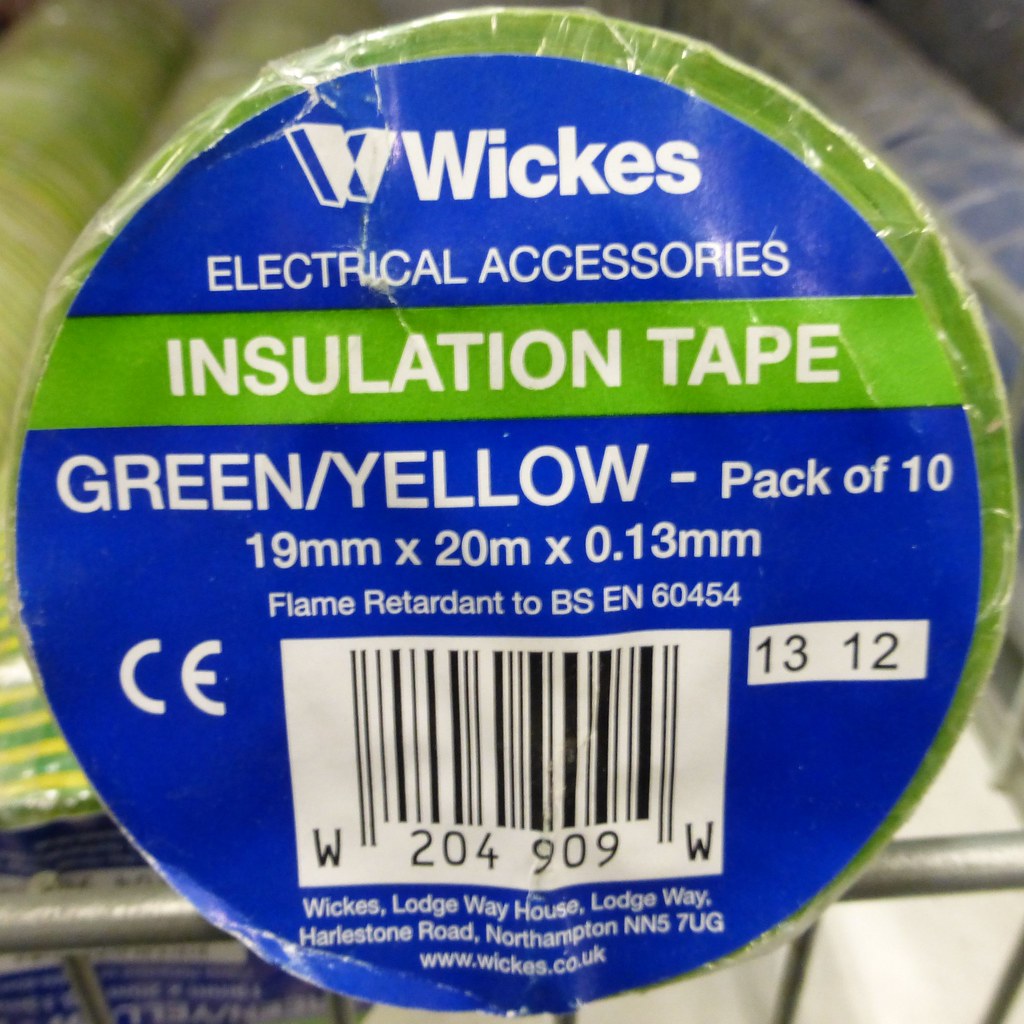This detailed photograph captures a green roll of insulation tape displayed at a store, likely a Home Depot or Lowe's. The tape has a circular blue label with white and green text. At the top of the label, there is a logo featuring an abstract 'W' with the brand name "WICKES" prominently displayed. The label reads "Wickes Electrical Accessories" in white text against a blue background. A lime green stripe with white lettering below it states "Insulation Tape." Further down, in white text against the blue background, it specifies "Green/Yellow Pack of 10," with dimensions listed as "19 mm x 20 m x 0.13 mm." The label also includes "Flame Retardant to BS EN 60454" and a barcode, accompanied by contact information including an address: "Wickes, Lodge House, Lodgeway, Harleston Road, Northampton, NN5 SUG, www.wickes.co.uk." The tape is packaged in a transparent wrapper, and the background of the image shows a blurred shelf, hinting at other rolls of tape.